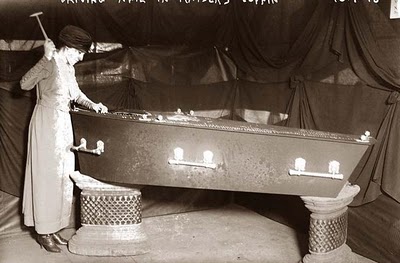In this antique-style, black-and-white photograph, we see a striking scene reminiscent of the late 1800s to early 1900s. At the center of the image is a woman dressed in period attire, donning a full blouse dress and a black hat. She stands poised with a small hammer raised in her right hand, evidently preparing to drive nails into the side of a coffin. The coffin, which appears to be made of metal, is supported by two ramshackle pedestals, one at each end, ensuring it remains upright for her task. This coffin also features three handles on its visible side, used by pallbearers in traditional funerary customs. 

Surrounding the scene is an array of black drapery, creating an ambiance of privacy and solemnity, with the dark fabric seemingly draped over a cold concrete floor. This setup suggests a makeshift private area, possibly within a larger building, with glimpses of windows partially obscured in the background. A stark light source spotlights the woman and the coffin, enhancing the dramatic and eerie atmosphere of the moment as she prepares to seal the coffin.